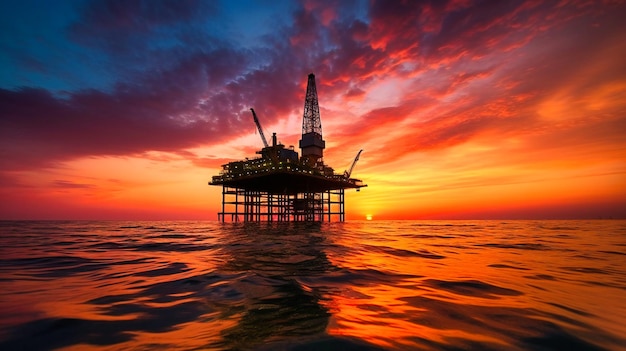In this photograph capturing either a sunrise or a sunset, a dramatic sky painted in brilliant shades of orange, red, and pink stretches across the horizon, transitioning to deep blues and purples in the top left corner. The ocean beneath is vast and calm, with only a few subtle ripples disturbing its surface. Dominating the scene is a solitary oil rig, silhouetted against the radiant backdrop. The structure, stationed in the middle of this expansive body of water, features a network of metal beams and scaffolding that form its support. A platform rests atop this frame, adorned with rows of yellow lights. Rising from the platform are cranes and towers, contributing to the intricate silhouette. The lack of surrounding features emphasizes the isolation of the oil rig in the vastness of the calm ocean waters.